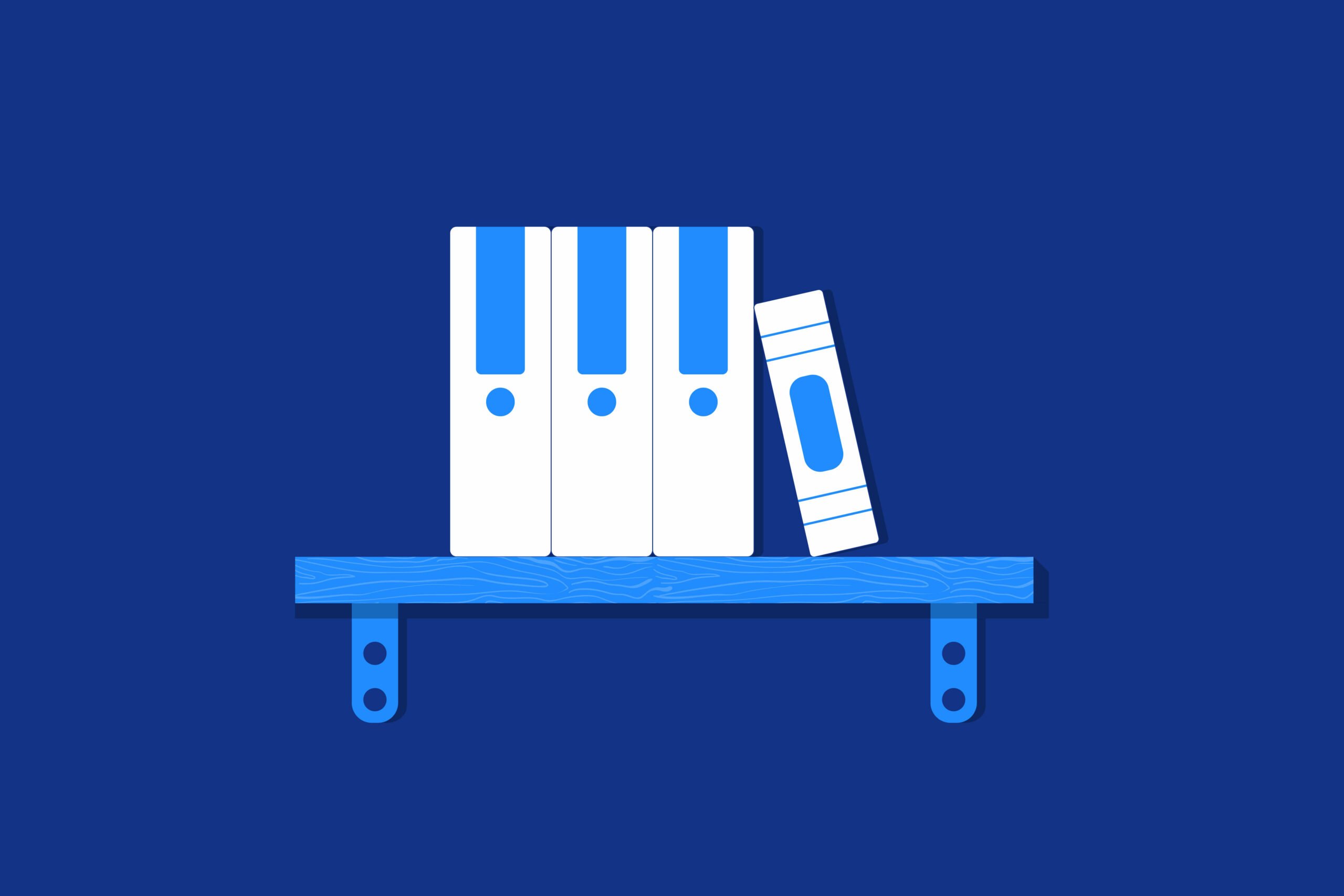The computer-generated illustration features a dark blue background with a centrally located light blue bookshelf secured to the wall by bolts. The shelf consists of a long narrow base with curved rectangular ends, each adorned with two circles. On the shelf, there are four books: three large white ones with light blue stripes and a central blue dot, all standing upright, and a smaller white book leaning against the trio. This smaller book has a blue pill-shaped stripe in the center and two horizontal blue stripes on either side. The overall scene is simple yet stylized, emphasizing minimalistic design and cohesive color coordination between the books and the shelf.